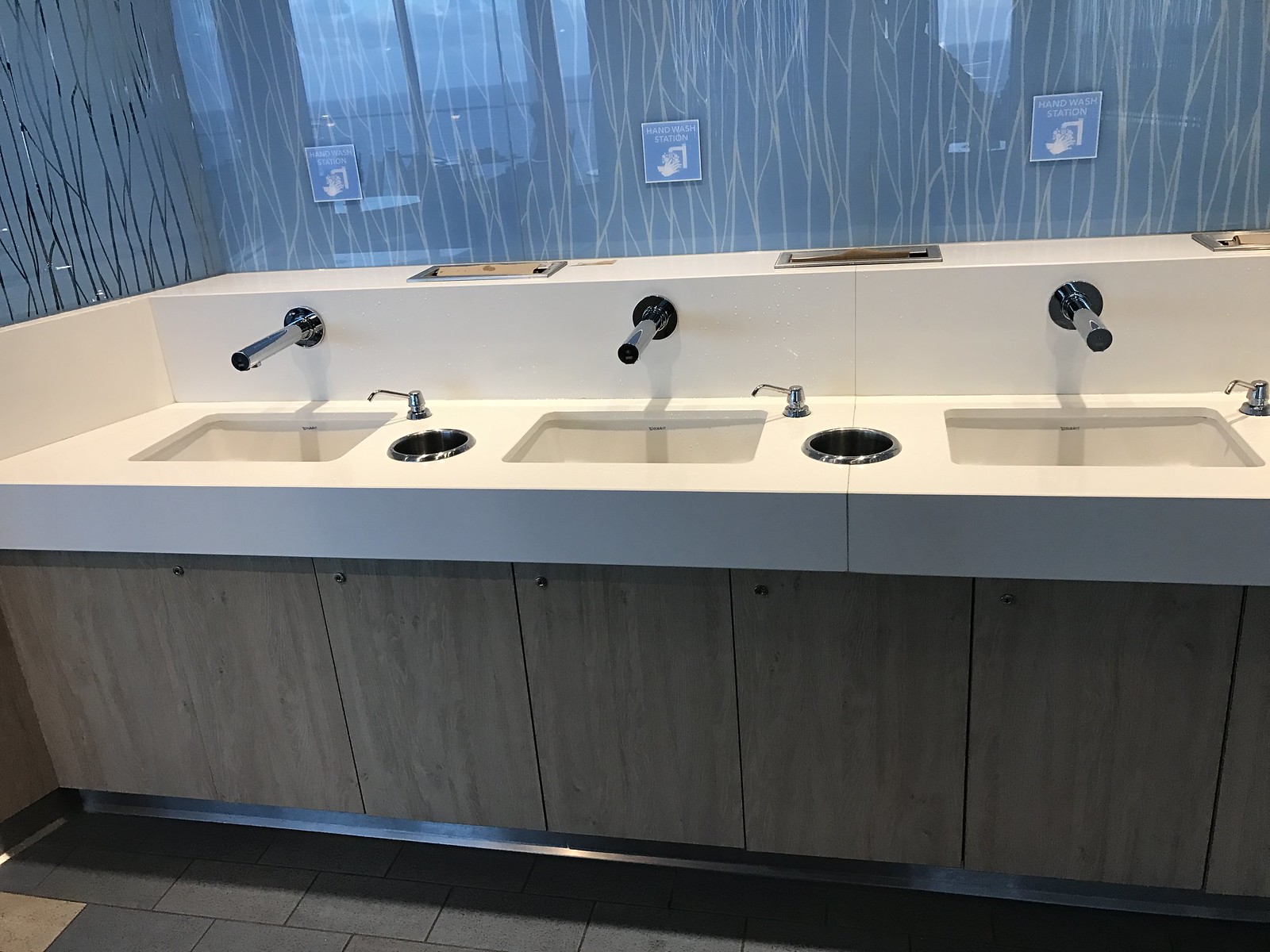The photograph captures a sleek, modern public restroom featuring three square, drop-in sinks set into a pristine white countertop. The surface below the sinks is adorned with gray, wood-grain cabinetry, lending a functional yet stylish appearance. Each sink is equipped with a modern, straight-tube faucet extending from the wall—likely motion-sensor activated—as well as a built-in metal pump soap dispenser. Discreet garbage receptacle holes are strategically placed between the sinks, seamlessly connecting to hidden bins behind the cabinet doors.

The bathroom's floors are adorned with elegant gray tiles, contributing to the overall clean and contemporary look. The walls behind the sinks are not mirrored but rather showcase a frosted glass backsplash with an intricate design resembling silver tree branches on a blue background. Above each sink, a sign reads "Wash Hand Station," accompanied by graphical instructions for proper handwashing. The cohesive design and thoughtful details emphasize both functionality and aesthetic appeal, suggesting that this restroom belongs to a large, well-maintained facility.